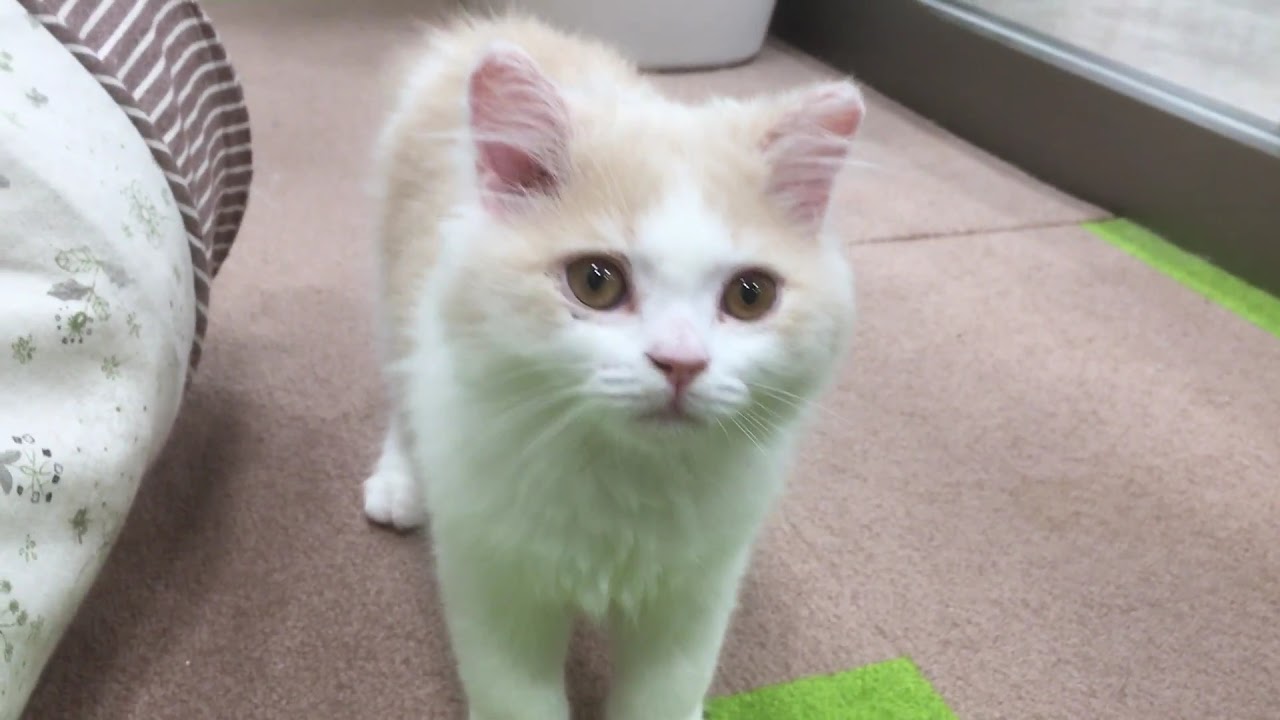This indoor photograph features a young white kitten with hazel eyes, light brown markings around its ears and body, pink ears, and a pink nose. The kitten is centrally positioned and is standing on a mostly pink carpet that has lime green accents along the edges. Adjacent to the kitten is a piece of cloth, possibly a blanket or bed covering, which is white with green floral patterns and brown accents. Behind the kitten, there is a white bucket. The backdrop includes a gray border, possibly indicating a wall or window. The mixture of colors in this detailed image includes shades of white, green, lime green, gray, pink, and brown.